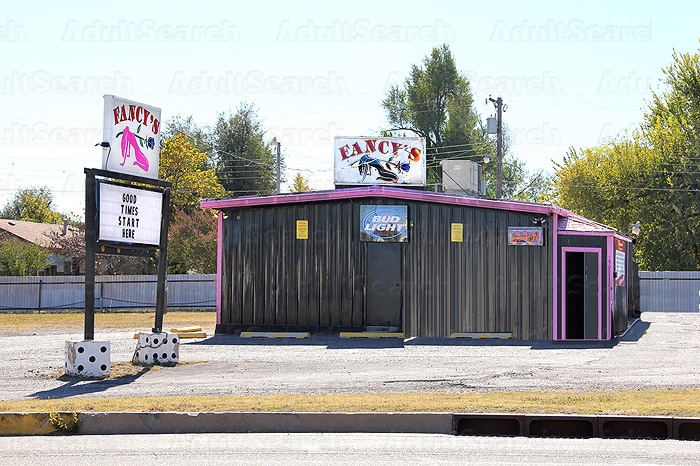This vibrant outdoor setting features a striking shop with a distinct pink roof and pink-framed door, set against a backdrop of lush green trees and a partly cloudy blue sky. The building, primarily constructed of dark brown wood with vertical grooves, proudly displays "FANCY" in bold red letters on a prominent sign atop the roof, accompanied by an illustration of a woman reclining with her hands pressing on the ground behind her.

To the left of the shop, a distinctive black sign supported by two dice-shaped bases, one showing five dots and the other six, declares "GOOD TIMES START HERE" in bold letters. The immediate surroundings include a parking lot devoid of cars, a white wooden fence separating the shop from the forested area in the background, and a house with a brown roof peeking through the trees.

At the front entrance of the shop, there is a black door with a rectangular Bud Light sign above it, displaying the brand name in white letters against a blue background. The trim of the building, including the door entryway and roofline, is painted in a vibrant pink that contrasts sharply with the dark exterior. To the right side of the building, there's a smaller section with purple trim and a red and blue "OPEN" sign. The overall scene is a colorful and inviting depiction of the business surrounded by natural beauty and clear skies.